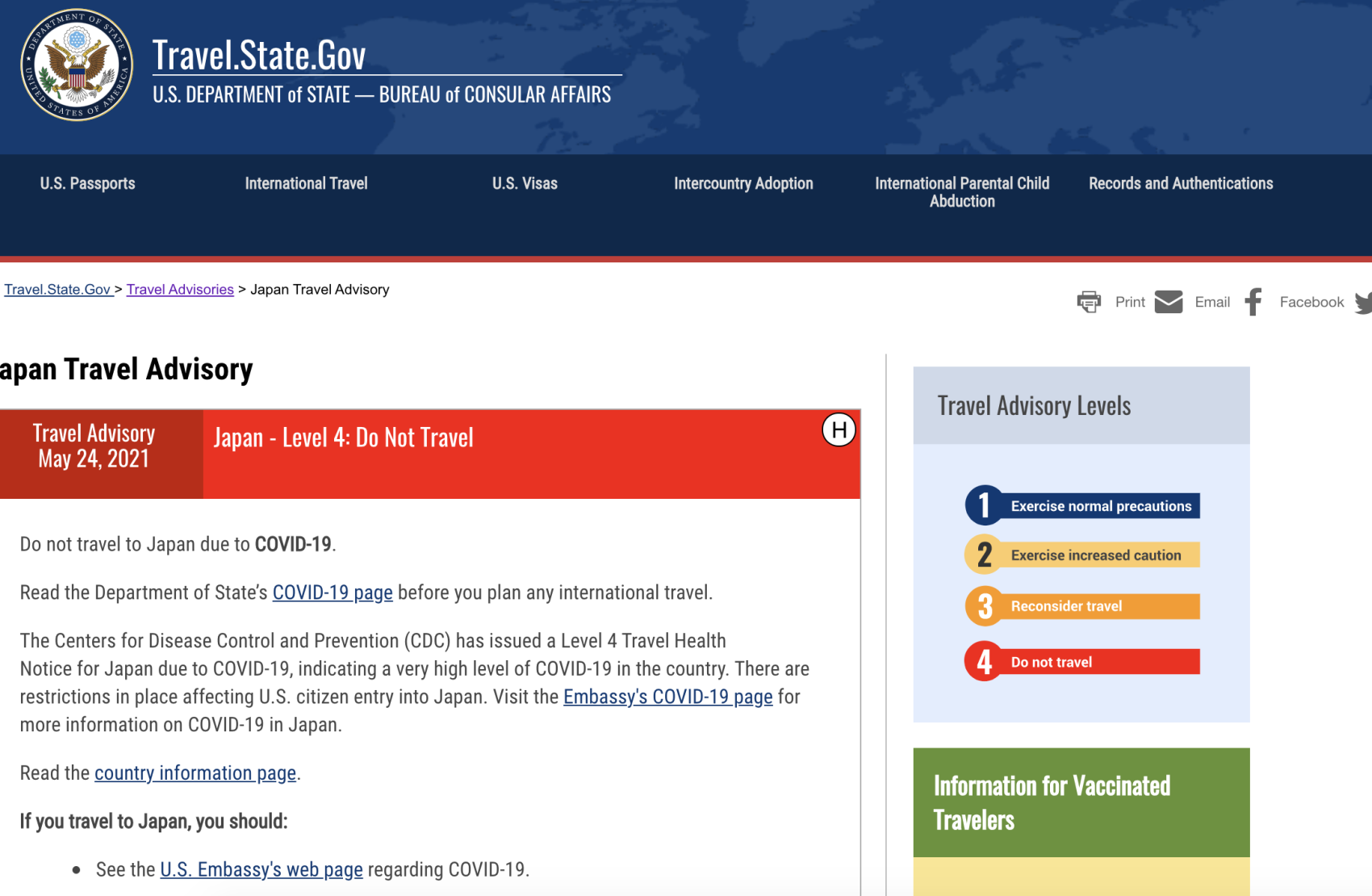The image depicts a government website, specifically travel.state.gov, under the U.S. Department of State, Bureau of Consular Affairs. Prominently displayed at the top is the official government seal featuring an eagle, situated to the left of the site’s title and departmental affiliation. 

Directly beneath this header, a range of navigation categories are listed, including options such as U.S. Passports, International Travel, U.S. Visas, Inter-Country Adoption, International Parental Child Abduction, and Records and Authentications.

The main section of the page features a prominent travel advisory for Japan dated May 24, 2021. The advisory categorizes Japan as Level Four: Do Not Travel, due to the COVID-19 pandemic. Visitors are urged to consult the Department of State's COVID-19 page before making any international travel plans. Supporting this advisory is a reference to the CDC's issuance of a Level Four travel health notice, with additional clickable links provided for more detailed information.

To the right, a color-coded chart is visible, serving as a key or legend to explain the different travel advisory levels. The chart is structured as follows: 

- Level One (dark blue): Exercise Normal Precautions
- Level Two (yellow): Exercise Increased Caution
- Level Three (orange): Reconsider Travel
- Level Four (red): Do Not Travel

Below this chart, there is supplementary information specifically for vaccinated travelers.